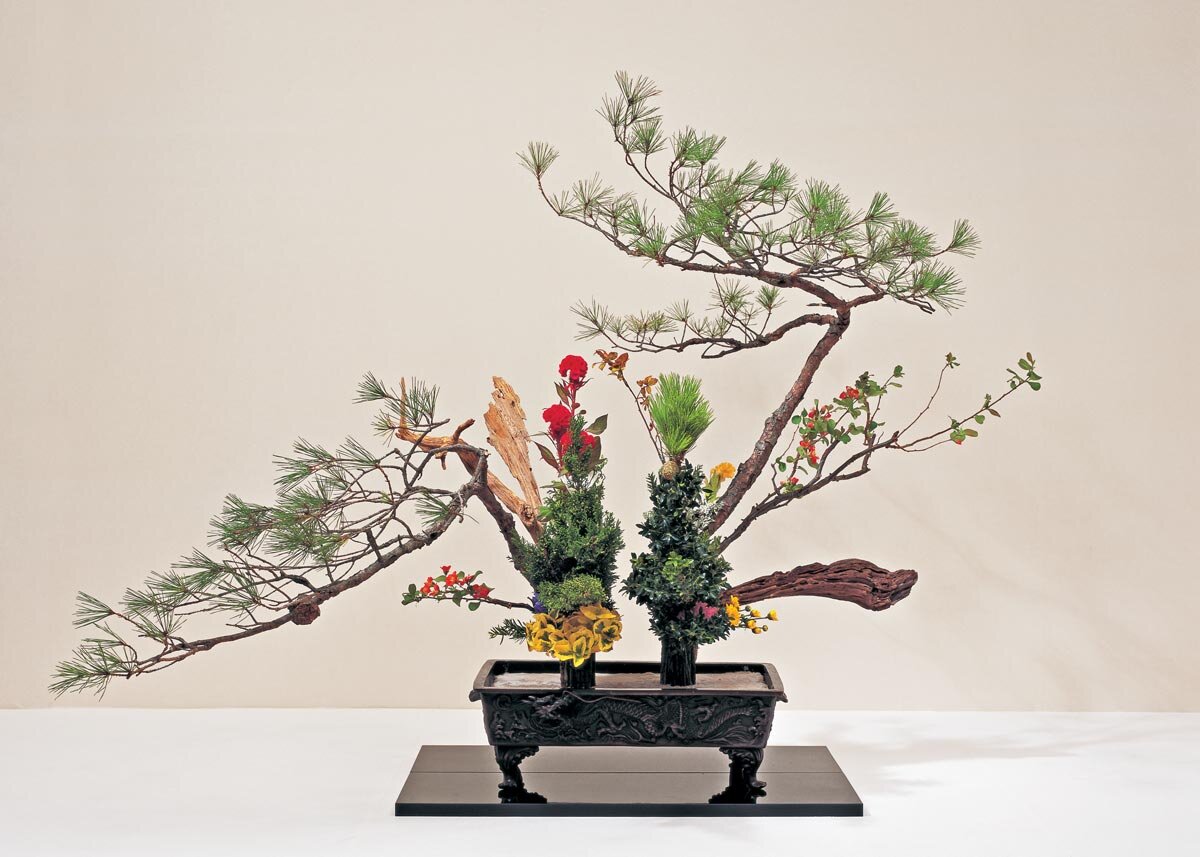This photograph showcases an elegant and intricately designed miniature table, which appears to be a sophisticated antique piece with ornate embellishments and two fancy legs. Resting on the black platform atop a white shelf set against a beige wall, the table holds two rectangular metal pots. Each pot contains miniature Japanese trees, reminiscent of tiny Christmas trees, complete with a delightful assortment of additional botanical elements such as bushes, leaves, and flowers. One pot features a tree with prominent branches that resemble pine needles, adorned with red flowers and yellow flowers at the base, interspersed with a beige and brownish branch. The second pot mirrors this arrangement with another miniature tree, decorated again with yellow flowers at the base and a large, errant branch stretching upwards. The overall effect is accentuated by what appears to be a painted backdrop, adding a further touch of abstraction and artistic charm to the scene.